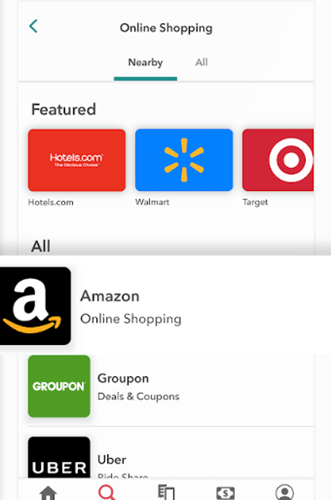This screenshot from a mobile device features a complex user interface set against a white background, indicative of an online shopping application. A prominent pop-up overlay partially obscures the underlying screen, adding to the layers of visual information. 

At the top of the screen, "Online Shopping" is displayed in bold text, accompanied by a back arrow button to facilitate navigation. Below this header, two tabs labeled "Nearby" and "All" are visible, with the "Nearby" tab currently selected. This section showcases a variety of thumbnail images representing different shops.

"Featured" is prominently displayed in black text beneath the tabs, followed by a series of recognizable brand logos, each accompanied by relevant text:

- **Hotels.com**: A thumbnail image indicates the presence of hotel booking options.
- **Walmart**: A blue thumbnail with the Walmart logo signifies its offerings.
- **Target**: A red thumbnail featuring the Target logo represents its online store.
- **Amazon**: Displayed in black text, the Amazon logo, with its distinctive white 'A' and curved yellow arrow, reads "Amazon Online Shopping" next to it.
- **Groupon**: A green square with "Groupon" in white text, alongside "Groupon Deals and Coupons."
- **Uber**: A black square with "Uber" in white text.

The bottom of the screen houses a navigation bar with a series of icons that provide quick access to different sections of the app:

1. **Home Icon**: Likely returns the user to the main page.
2. **Magnifying Glass/Search Icon**: Opens the search function.
3. **Copy Icon**: Could be associated with saved or copied deals.
4. **Money Icon**: Probably related to payment options or deals.
5. **AdWords Profile Icon**: Presumably links to user profile or advertisements.

Overall, the image captures a detailed, multi-functional interface designed to streamline online shopping and access to various services and deals.